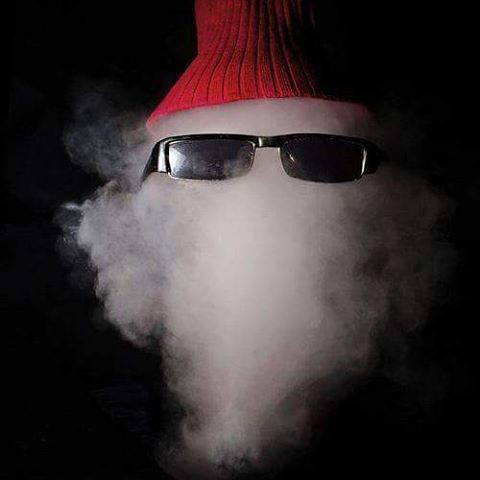The photograph depicts a cleverly arranged scene where a billowing cloud of white smoke or possibly cotton is shaped to resemble a bearded face, somewhat reminiscent of Santa Claus. The main features of this anthropomorphic creation include a pair of black sunglasses partially enveloped in the "beard" formed by the smoke or cotton, positioned where eyes would typically be. Atop this whimsical face, a red knit beanie is placed as a hat. The puffy white "beard" extends down into a V shape and spreads out to the sides, creating a bushy effect. The entire composition is lit against a completely black background, emphasizing the ghostly yet festive figure emerging from the darkness.